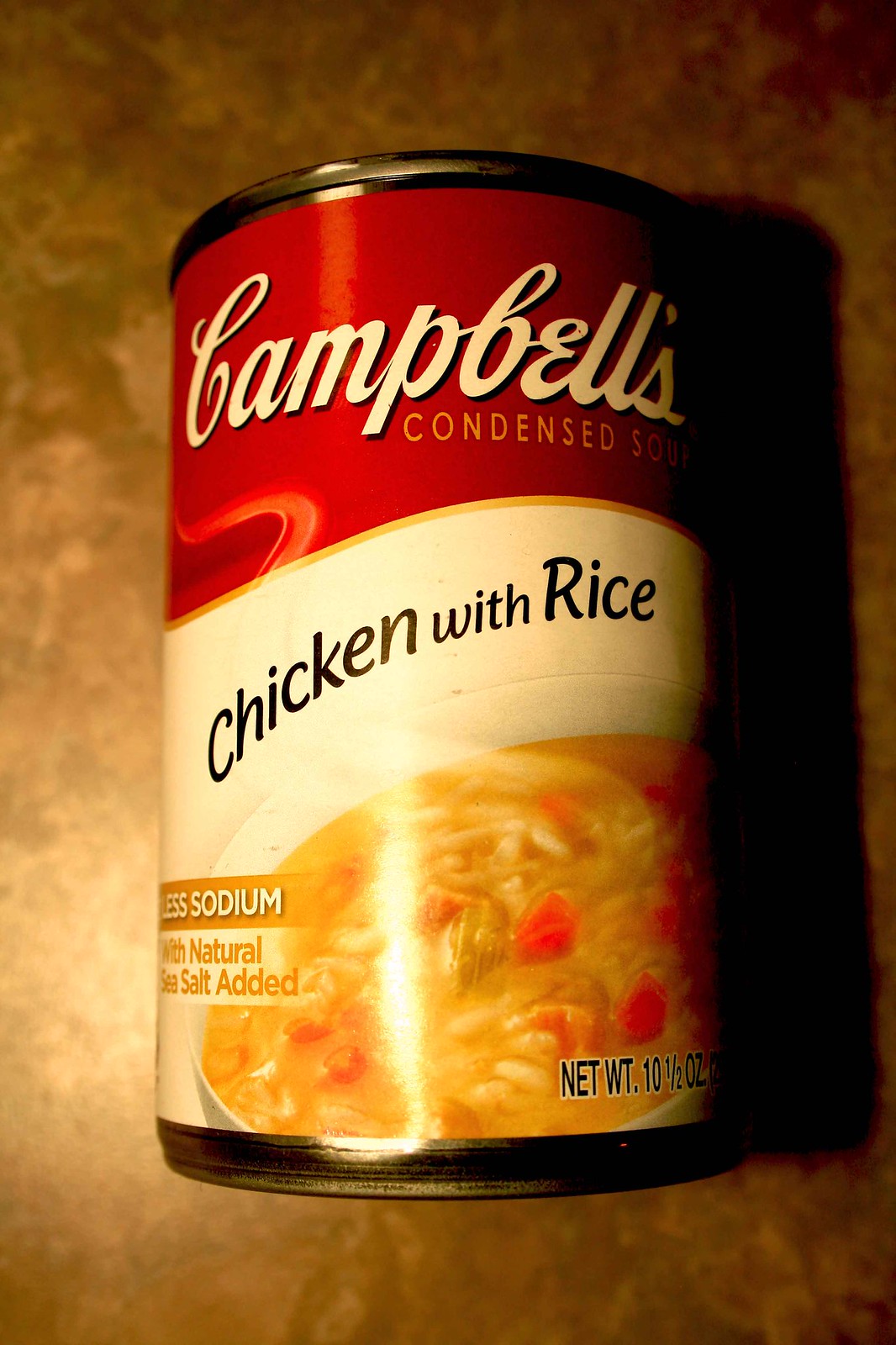This is a close-up photograph of a Campbell's Condensed Soup can, specifically the Chicken with Rice flavor. The can is made of aluminum and is laying on its side on a glossy, goldish-brown marbled countertop. The image was taken with a flash, causing a bright glare on the front of the can and creating a harsh shadow against the dark background. The label consists of a red top half, featuring the iconic Campbell's cursive logo in white, and a white bottom half with black text stating "Chicken with Rice." Below the text, there's a detailed, close-up image of a bowl of the soup, which shows visible grains of rice, and small bits of carrot and possibly celery. There are also two banners on the label: one on the bottom left in white text on an orange-yellow background that reads "Less Sodium," and another on a white background with orange-yellow text declaring "With Natural Sea Salt Added." The bottom right of the label, partially obscured as it curves around the can, indicates the net weight of 10.5 ounces.